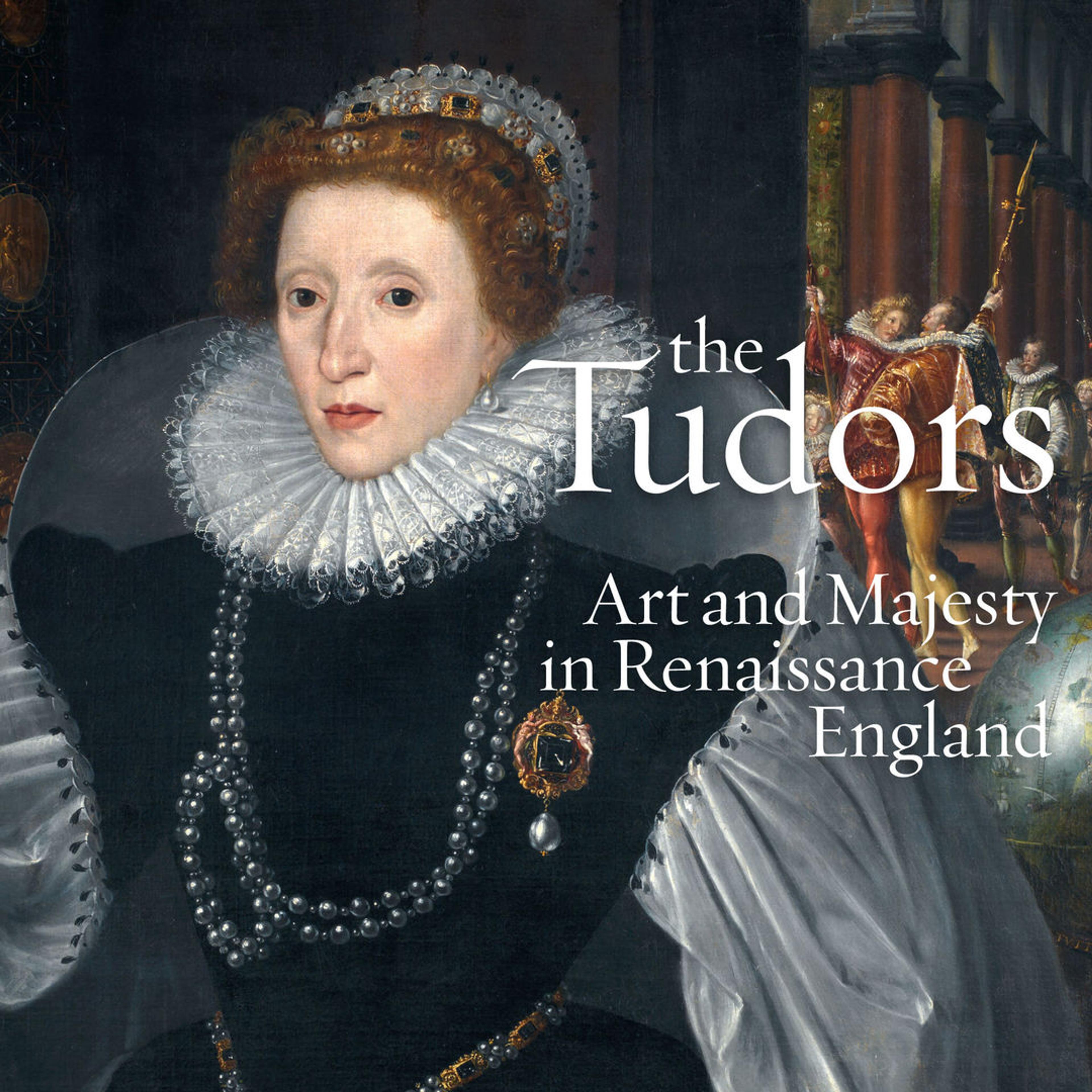This detailed painting captures a regal woman, possibly Queen Elizabeth I, dressed in full Renaissance attire. She has striking red hair, a very pale complexion with pink lips, and is adorned with an opulent white crown. The text to the right of her reads "The Tudors: Art and Majesty in Renaissance England," adding context to the era and significance of the artwork. 

The woman is facing slightly to the left but predominantly looking forward. She is enveloped in a grand, black gown adorned with black pearls or a string of onyx around her neck. The gown includes an elaborate neck piece that fans out around her head and down to her shoulders. Her voluminous sleeves, which appear to be silver or possibly white with gray undertones, puff out dramatically before cinching at the waist, which is encircled by a slender gold and blue belt.

Her outfit is further accentuated by intricate jewelry, including a notable brooch pinned on her left breast, featuring a central gemstone and a dangling Tahitian pearl or silver ball. Behind her, the backdrop consists of a plain black wall which gives way to a vibrant scene. To her right, beyond the text, there are figures dressed in rich, extravagant colors such as reds, oranges, and greens, with some men holding spears and dancing amidst grand columns, which adds a layer of depth and opulence to the historical setting.